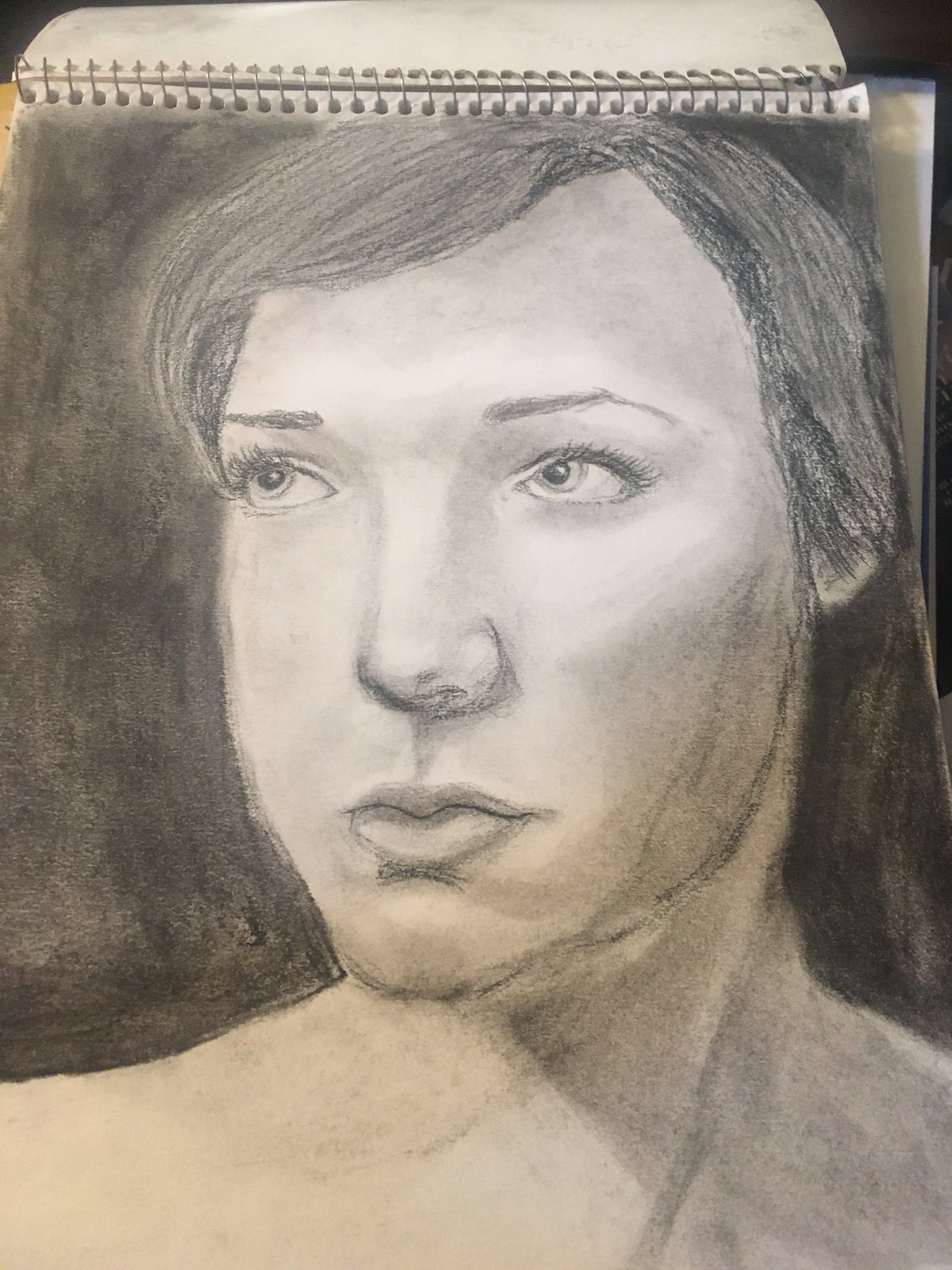This image captures a hand-drawn portrait of a young woman, executed in either pencil or charcoal on a sketch pad still attached to a binder, indicated by the visible metal rings at the top. The artist, likely a burgeoning talent, has depicted an oval-shaped face with thin eyebrows, expressive eyes looking up and to the left, and a normal-shaped nose and lips. The woman's grayish-brown hair appears short, partially covering her right earlobe and cheekbone. She has no shirt on, revealing just the top of her shoulders and neck. The background is a dark gray, blending somewhat with her hair, and there's prominent shading and shadowing on her face, contributing to her solemn, slightly sad expression. The drawing is monochromatic, with no additional writing or colors present.